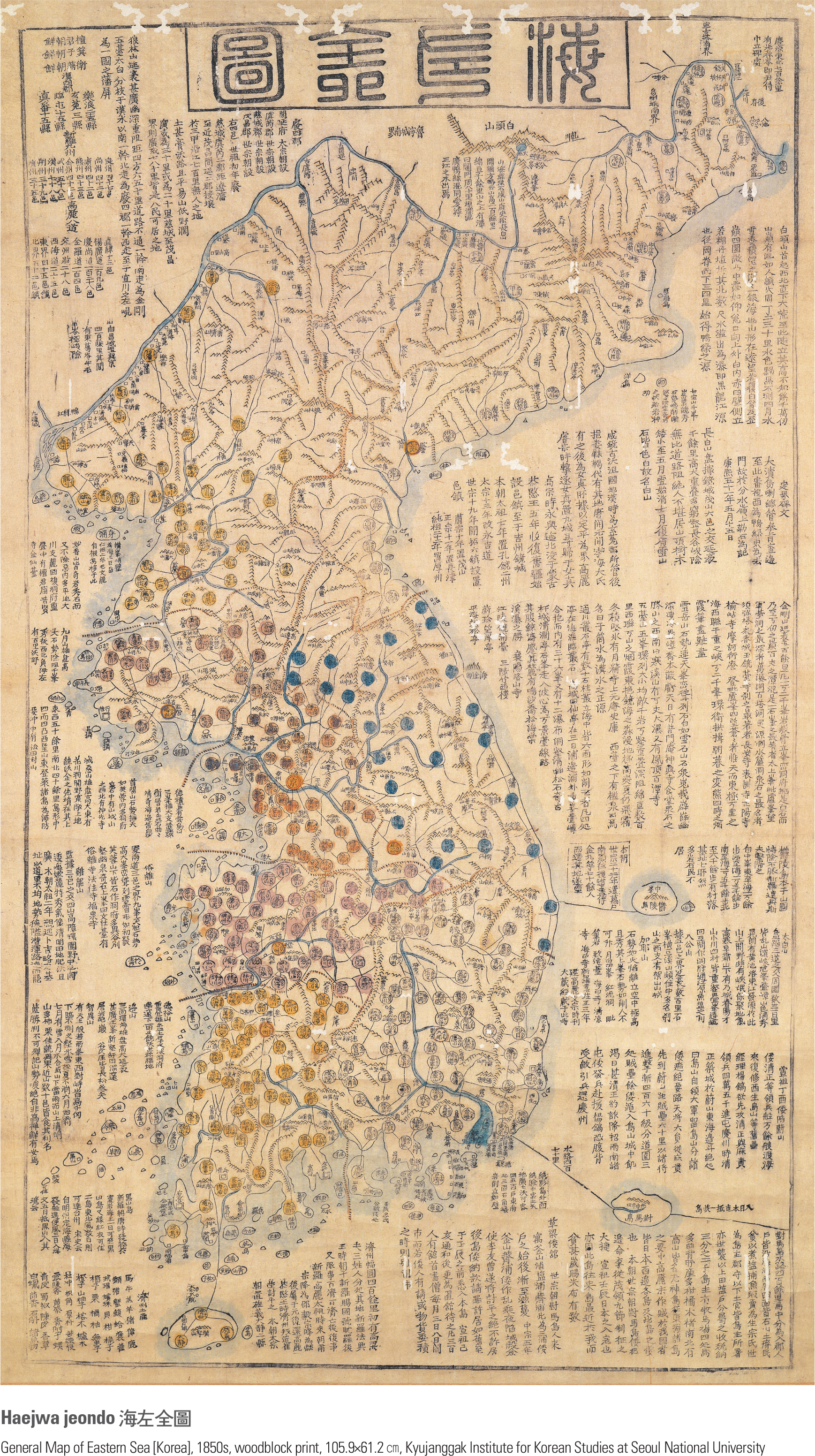The image depicts a beautifully detailed, rectangular map on faded brown paper, showcasing an island or part of a country, surrounded by water. Dominated by text in an Asian language, likely Japanese or Korean, the map is adorned with vertical and horizontal script, with four prominent Asian characters at the top and circled text on the sides. Blue, yellow, and pink dots sprinkle across the central geographic landmass, potentially indicating significant locations or features. Stylized squiggle lines, possibly detailed borders, rivers, or roads, scatter the upper region. The map is bordered by a black line and, at its bottom, contains English text. This text reads "Heijowa Jeondo, General Map of Eastern Sea, Korea, 1850s," with a note crediting the print as produced by the Institute for Korean Studies at Seoul National University.